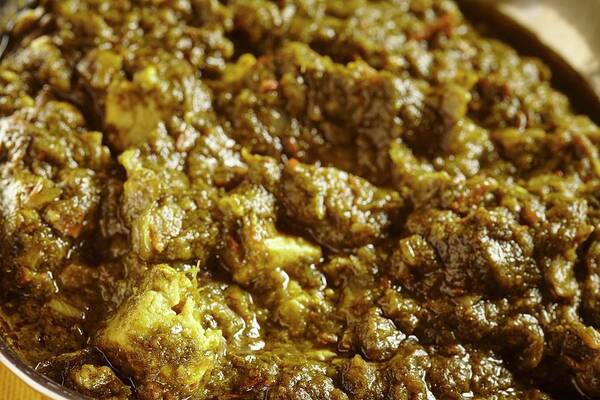This image features a close-up view of a food dish, likely a green curry, presented in a container that appears to be either ceramic or metallic with a subtle curve visible at the upper right and lower left corners. The dish itself is a chunky, greenish-yellow colored curry with distinct thick gravy. It contains visible cauliflower florets, pieces of meat or vegetables, and small bits of orange that may be peppers, giving some diversity in texture and color. The curry's consistency varies, appearing thicker on the cauliflower while maintaining an oily, soupy texture in other areas. The surrounding context is minimal, with only a hint of a wooden counter at the very left-hand corner of the image.